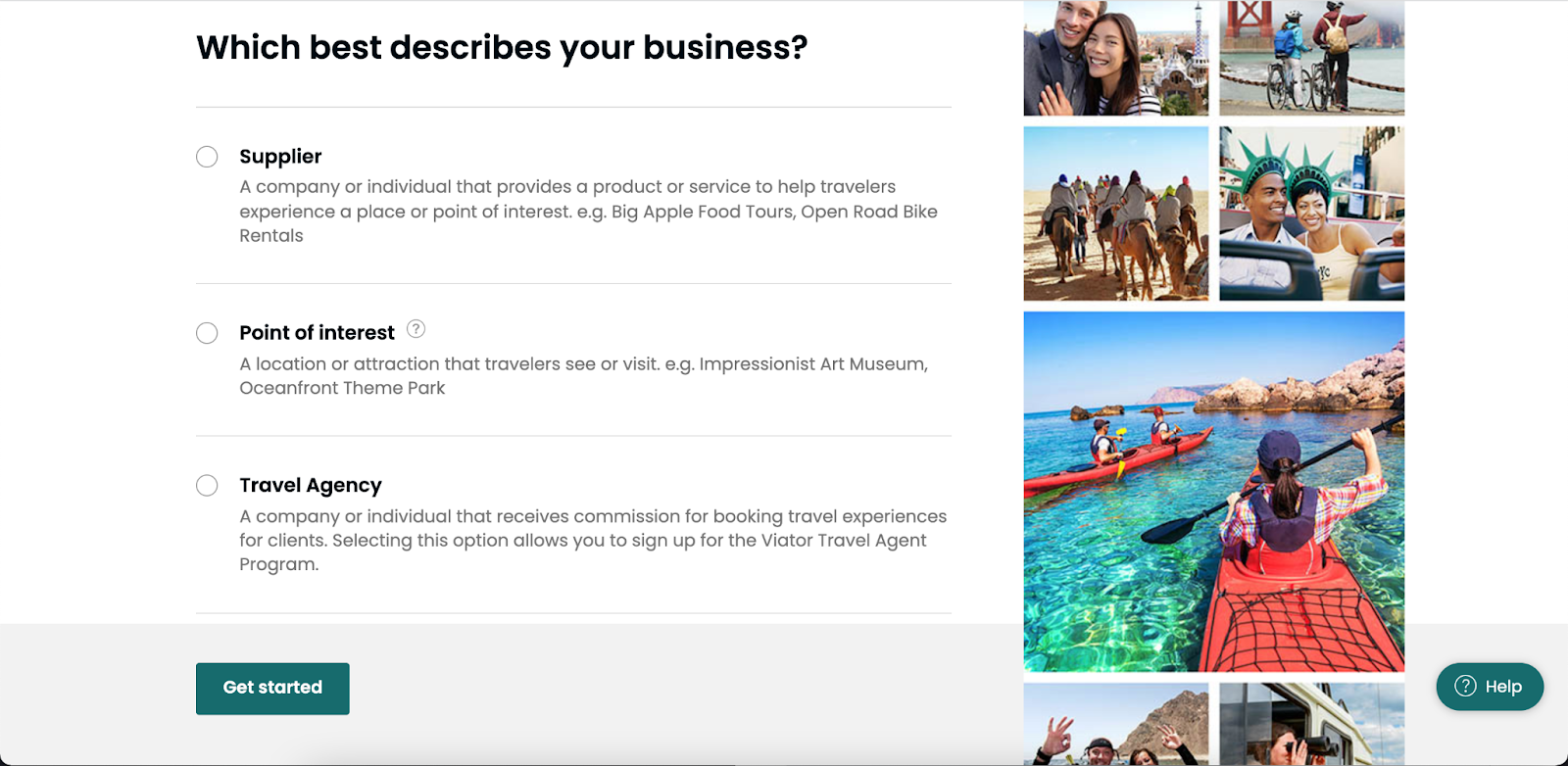The webpage features a clean white background with black font aligned to one side, creating a crisp and professional layout. The text header reads, "Which best describes your business?" followed by a series of selection options, each accompanied by a circular checkbox. 

1. **Supplier**: Described as a company or individual that offers products or services aiding travelers in exploring destinations, such as "Big Apple food tours" or "Open road bike rentals."
2. **Point of Interest**: Defined as a specific location or attraction that tourists visit, like an "Impressionist Art Museum" or an "Oceanfront theme park."
3. **Travel Agency**: Identified as an entity that earns commissions by booking travel experiences for clients. Clicking this option prompts a sign-up for the "Vic Viator travel agent program," accompanied by a teal button labeled "Get Started."

On the opposite side of the webpage, various images are displayed:

- A smiling brunette-haired woman and a man; she rests her hand on his chest while wearing a white and black striped shirt, and he is dressed in gray.
- Two individuals biking with the Golden Gate Bridge visible in the background.
- Several people, possibly on horseback or camels, dressed predominantly in gray.
- A smiling African-American couple donning playful, green Statue of Liberty-like hats.
- People paddling red kayaks on a turquoise-green body of water.

At the bottom, two smaller, cropped images are visible:

- A man and a woman making the 'okay' hand sign, appearing joyful.
- A woman using binoculars.

The layout is completed with another teal and white box labeled "Help" at the bottom.